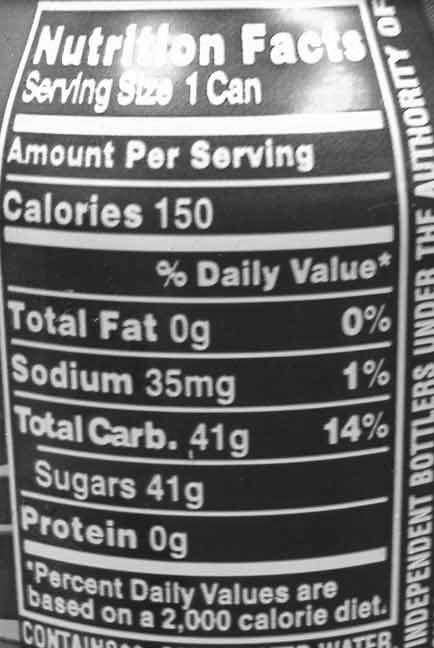This close-up photograph vividly captures the back of a black can, focusing on its nutritional label. The label, framed by a white outline, is predominantly black with white text. Starting with "Nutrition Facts," the label specifies a serving size of one can, detailing an amount per serving of 150 calories. The listed nutritional values include total fat at zero grams (0%), sodium at 35 milligrams (1%), total carbohydrates at 41 grams (14%), sugars at 41 grams, and protein at zero grams. An asterisk next to the percentage daily values indicates these are based on a 2,000-calorie diet. Additionally, to the right of the label, partially visible text reads, "independent bottlers under the authority of," though it is cut off. The angle reveals the faint slope of the can's top, confirming its form.